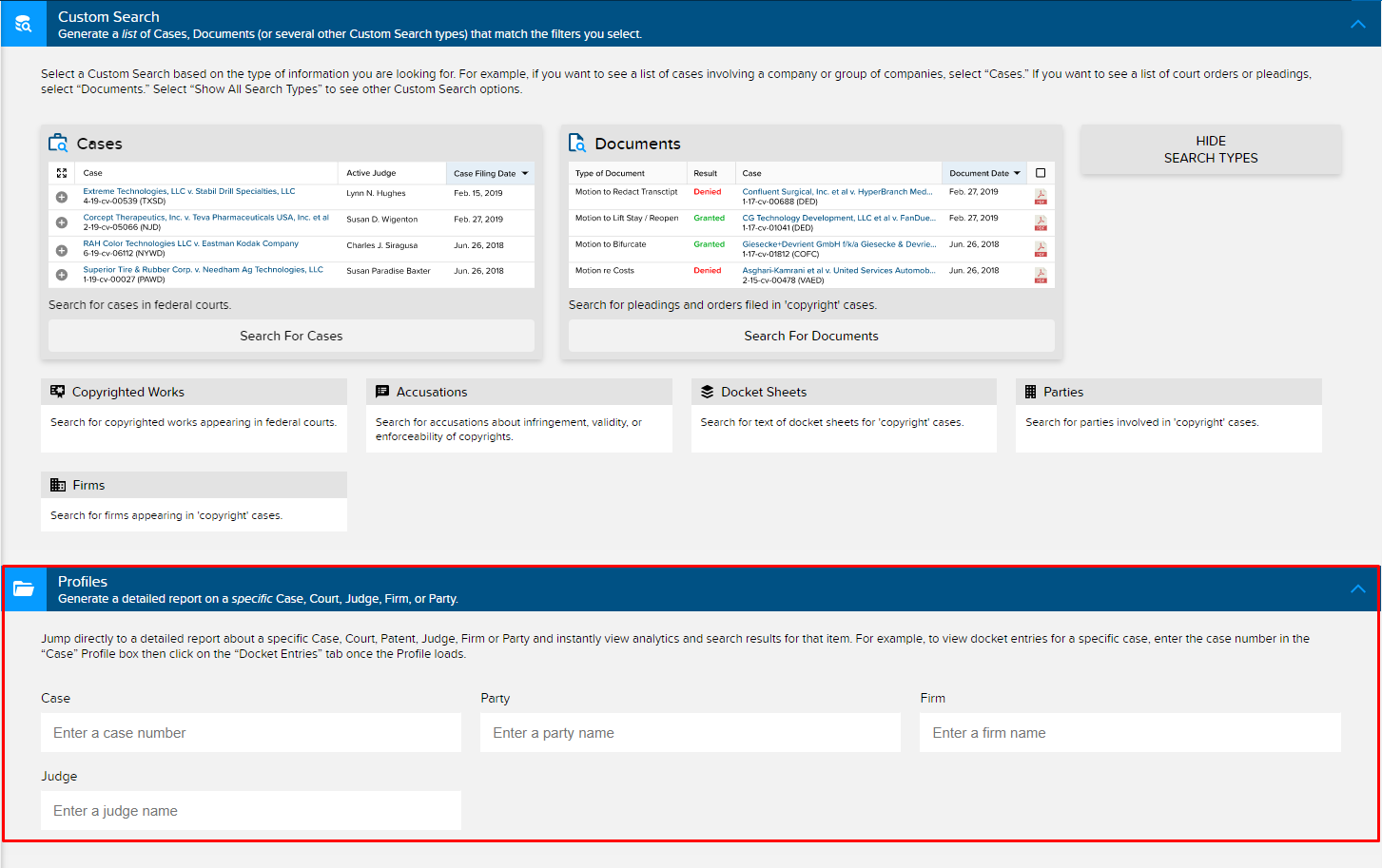The image depicts a custom search interface for what appears to be a public court records website. At the top, the title "Custom Search" is prominently displayed, though there's no visible web address to identify the specific site. The main section of the page provides instructions for generating various lists of cases, documents, or other search types based on user-selected filters. 

The instructions detail how to conduct a custom search. For example, users aiming to search for cases involving a company or a group of companies are advised to select the "Cases" option. To view court orders or pleadings, users should opt for "Documents."

On the left side of this interface, there are two primary menus. The first menu is labeled "Cases" and lists specific cases such as "Extreme Technologies vs [Unidentified] Specialties," along with four additional cases. These cases have filing dates ranging from 2018 to 2019. To the right of this, the "Documents" section features a dropdown menu offering options to filter by document type, result, case, document, and date. An example given here is a "Motion to Redact Transcript," which is noted as "Denied."

Further to the right, there is a clickable option labeled "Hide Search Types." Below this section, various categories like "Copyrighted Work," "Accusations," "Docket Sheets," "Parties," and "Firms" are listed.

At the bottom of the interface, there is a red-bordered box labeled "Profiles," which indicates users can create a detailed report on a specific case, court, judge, firm, or party. Users must input the relevant case, party, firm, and judge information to generate these detailed reports. This feature appears designed to provide comprehensive information about the selected legal entities or proceedings.